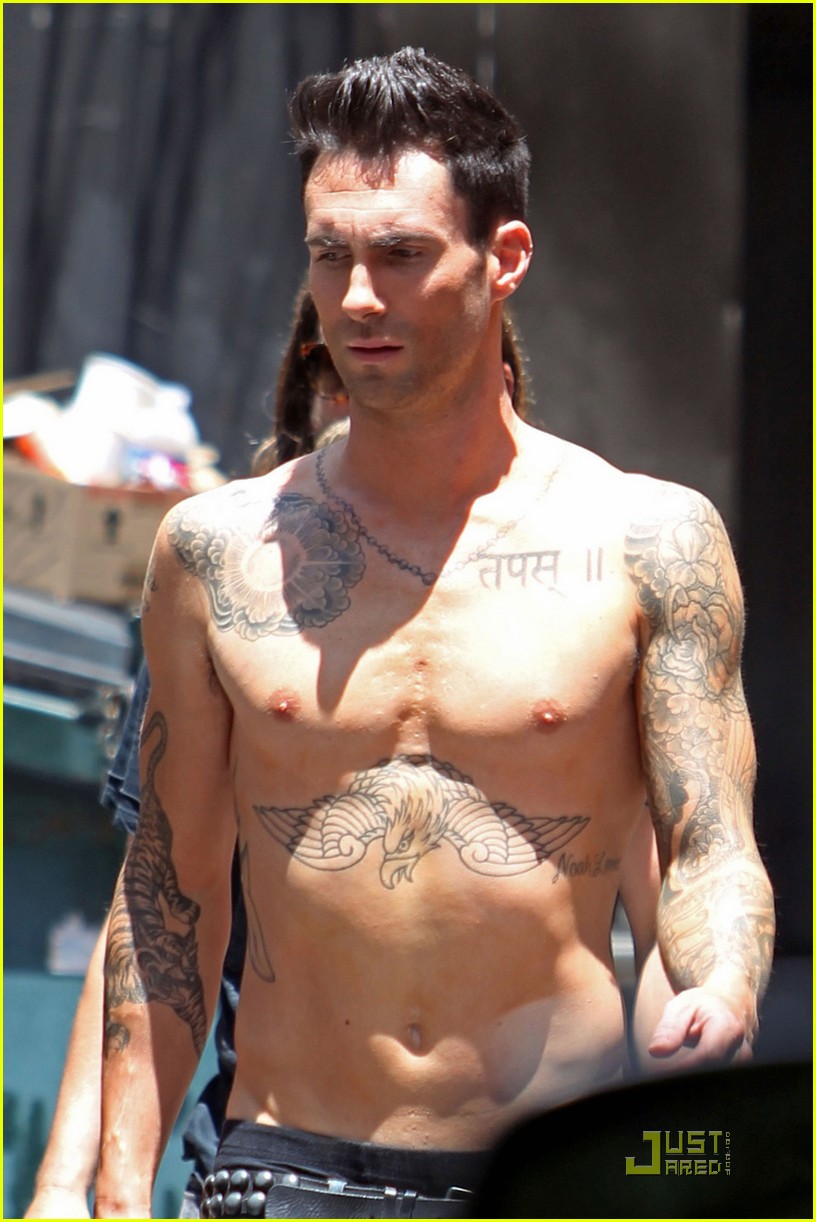In this highly detailed image, Adam Levine is captured standing shirtless outdoors under a sunlit sky. His outfit consists of black pants accompanied by a black studded belt. His numerous tattoos are prominently visible, including an eagle diving tattoo below his chest, a black tiger tattoo on his right arm, and a series of roses on his left arm. His other notable ink comprises a flower tattoo on his right shoulder, and what appears to be a necklace tattoo around his neck. He has short, brushed-back brown hair, no facial hair, and appears focused with his head slightly turned to the left. Behind him stands a woman wearing sunglasses, but her features are indistinct. Further in the background on the left, there is a cardboard box on a surface that might be a dumpster, filled with nondescript materials. A dark curtain or wall forms part of the backdrop. In the bottom right corner of the image, a yellow-lettered logo reads "Just Jared."